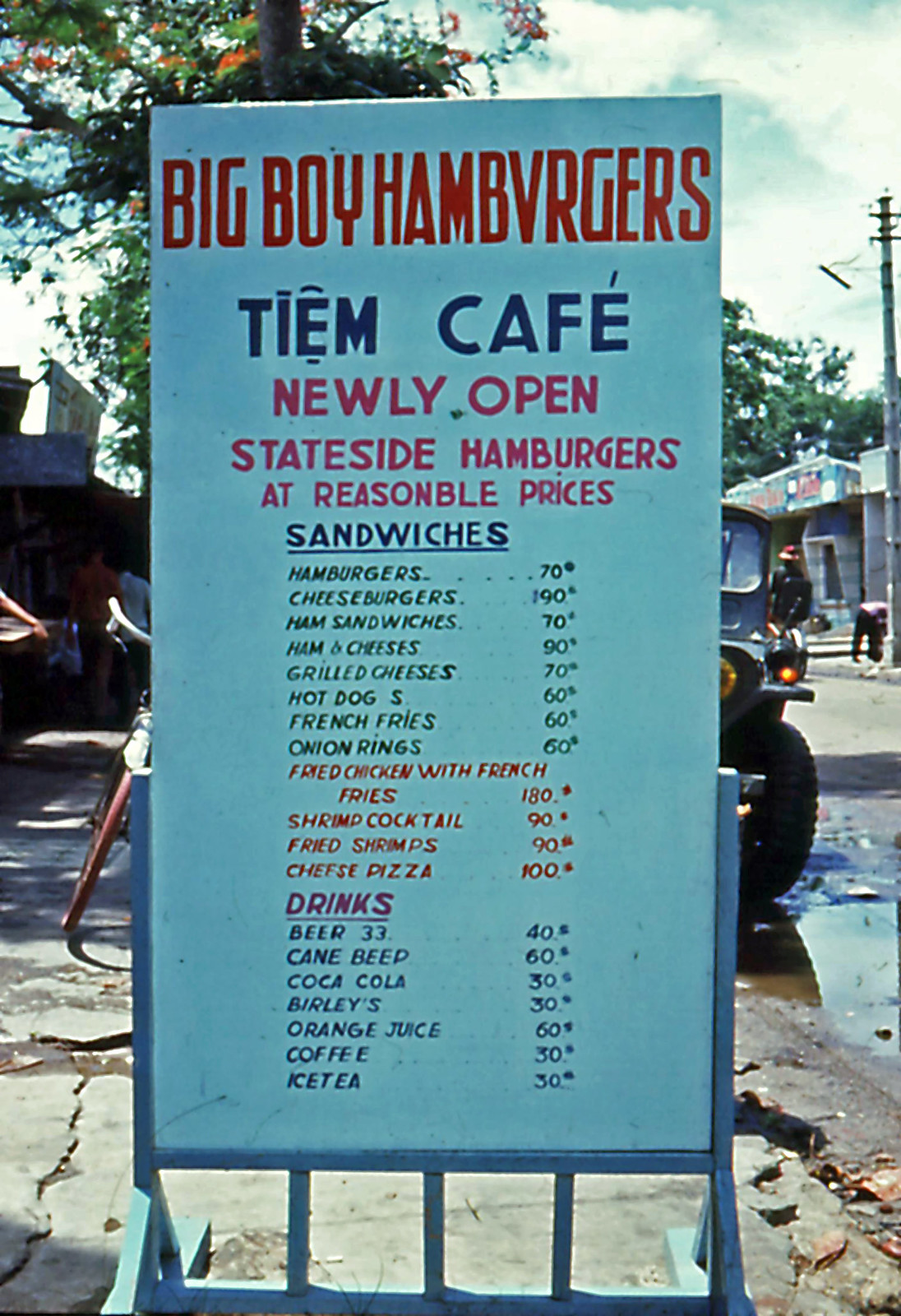In the image taken outdoors, a café menu is prominently displayed on a whiteboard framed in light blue, supported by a structure resembling a sideways ladder. The frame includes crossbars laying flat on the ground, angled uprights, and additional support bars.

In the background, broken concrete and water can be seen, along with the left side of a blue Jeep. The Jeep's front tire, fender, and part of the windshield are visible behind the sign. A green deciduous tree is on the left side, while more trees and various wires are seen towards the upper right side of the image.

A person, slightly bent over, stands near a pole, while another individual wearing what appears to be a Santa Claus hat walks along the street. The backdrop includes buildings with flat roofs, featuring windows with protective shutters against the sun. One building, light blue with a darker blue stripe and green and red writing on the top, adds to the scene.

A bicycle leans against the left side of the sign, revealing its front wheel, fender, and part of the handlebars. An arm is also visible on the left side. 

The menu advertises "Big Boy Hamburgers" with a unique presentation. Items listed include burgers, sandwiches, hot dogs, fries, onion rings, fried chicken, shrimp cocktail, pizza, drinks, beer, Coca-Cola, Burley's, orange juice, coffee, and ice cream. The café highlights its newly opened status and promises reasonable prices.